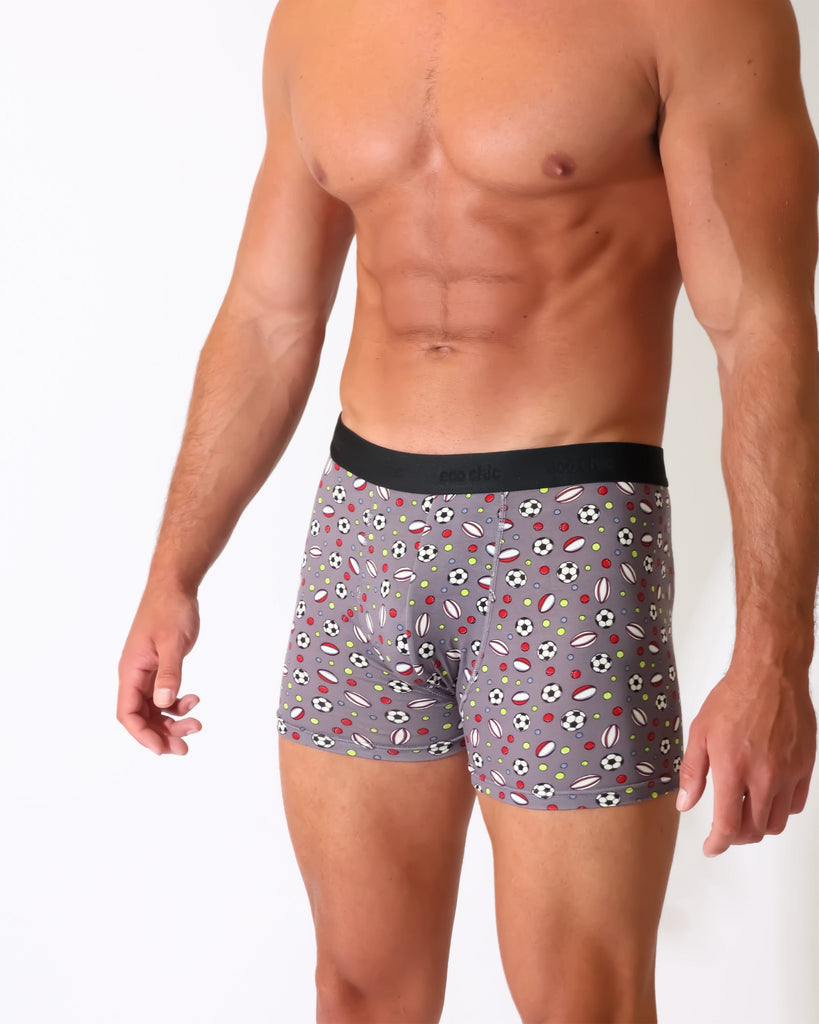This digital photograph showcases a well-toned, fit man from his chest down to just below his knees, posed while modeling a pair of boxer briefs. The man's skin has a darker tone with a nice tan, emphasizing his defined six-pack abs and muscular arms that hang naturally by his sides. His thighs also appear muscular.

The boxer briefs feature a prominent black waistband. The primary color of the briefs is gray, adorned with a playful and ongoing pattern of various sports balls, including black and white soccer balls, red and white footballs, tennis balls, rugby balls, and possibly smaller golf balls. There are also hints of yellow and blue accents amidst the pattern. The mixture of these elements creates a dynamic and eye-catching design on the underwear. Overall, there are no other objects or text in the image, making the focus solely on the man and the detailed design of the boxer briefs he is modeling.